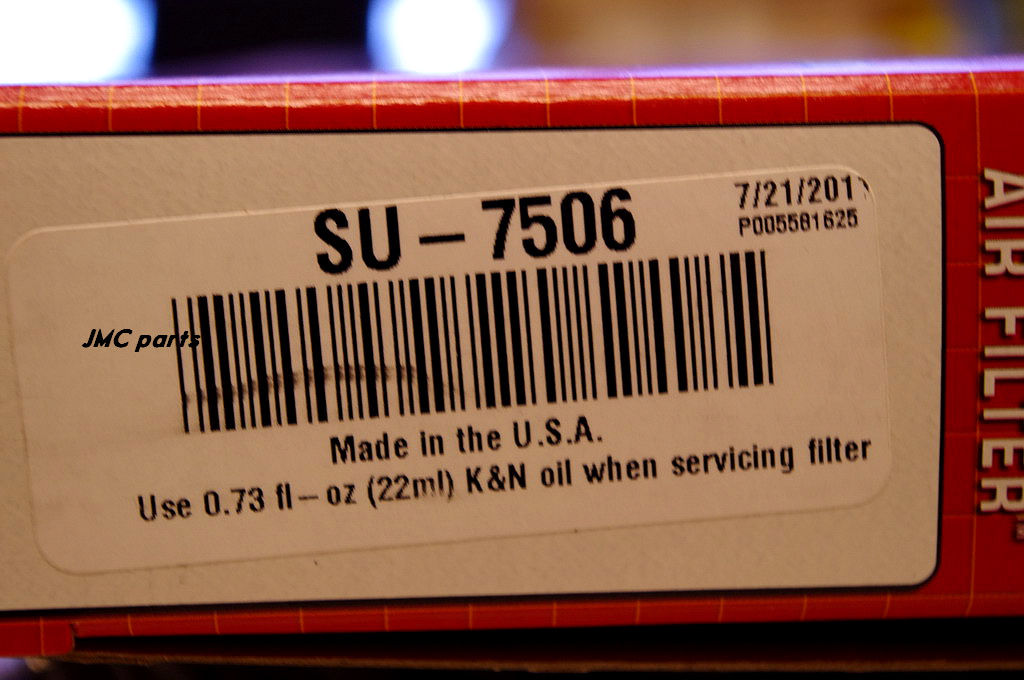The photograph features a close-up of the side of a red air filter box, prominently displaying the words "air filter" in white. The box has yellow striping and a detailed label at its center. The label includes a prominent serial number, "SU-7506," above a black and white barcode. Below the barcode, it reads "Made in the USA," and provides servicing instructions that specify the use of "0.73 FL-OZ (22 milliliters) K&N oil." The top right of the label shows a date as "7-21-20–," with the final digit faded and unclear, possibly indicating a year in the 2010s. The air filter is identified as a product of JMC Parts.